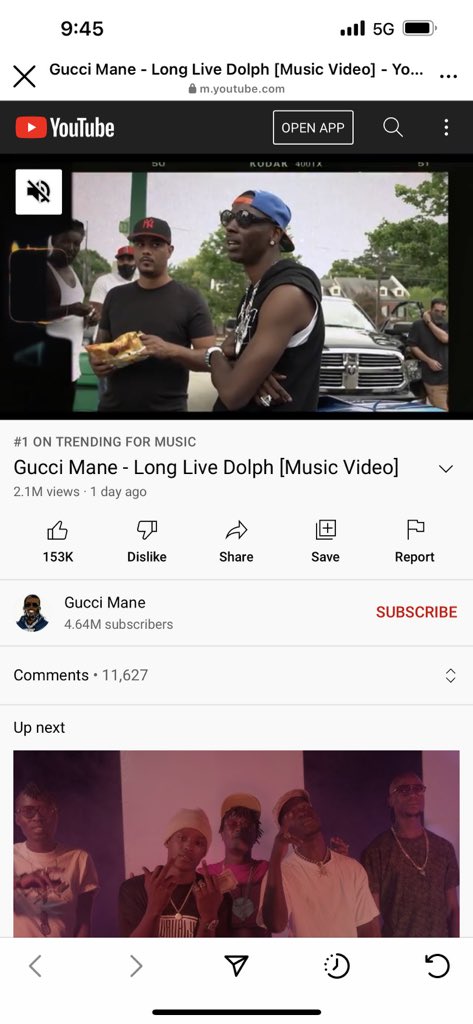A close-up screenshot of a smartphone screen displaying the "Long Live Doll" music video by Gucci Mane. The video is currently trending as the number one music video, with 4.64 million subscribers on the artist's channel. The view count shows 1,530,000 views, and it has a significant number of likes but also notable dislikes. Options to share, save, and report the video are visible beneath the video player. The top of the screen shows a full 5G signal and full battery icon. The pictured screen includes a fine glass Square device. On the right side of the screen, there are icons for left and right navigation arrows, a circle refresh button, and an area at the bottom identified as the supposed black bar.